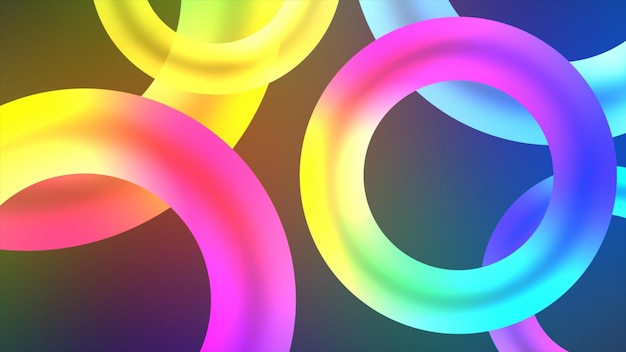This image showcases a visually striking collection of neon-colored circles against a dark background. Six rings are distributed across the image, each varying in visibility and color. 

In the bottom left corner, a large ring prominently features a vibrant mix of hot pink and yellow. Behind it, a slightly transparent ring displays shades of pink, yellow, and green, partially obscured by the foremost ring. Moving upward, an almost entirely visible gold or yellow ring extends from the top left.

On the right side of the image, at the top, a cyan ring partially emerges from the edge, only half visible. Below it, another ring displays cyan and lighter blue hues, partially hidden from view. Dominating the bottom right quadrant is a multicolored circle that blends pink, blue, green, and purple, beside which lies a three-quarters visible ring accented with pink, blue, and green tones.

The detailed layering and rich hues of the rings, coupled with their partially overlapping positions, suggest a captivating depth and dynamic composition, likely computer or AI-generated.